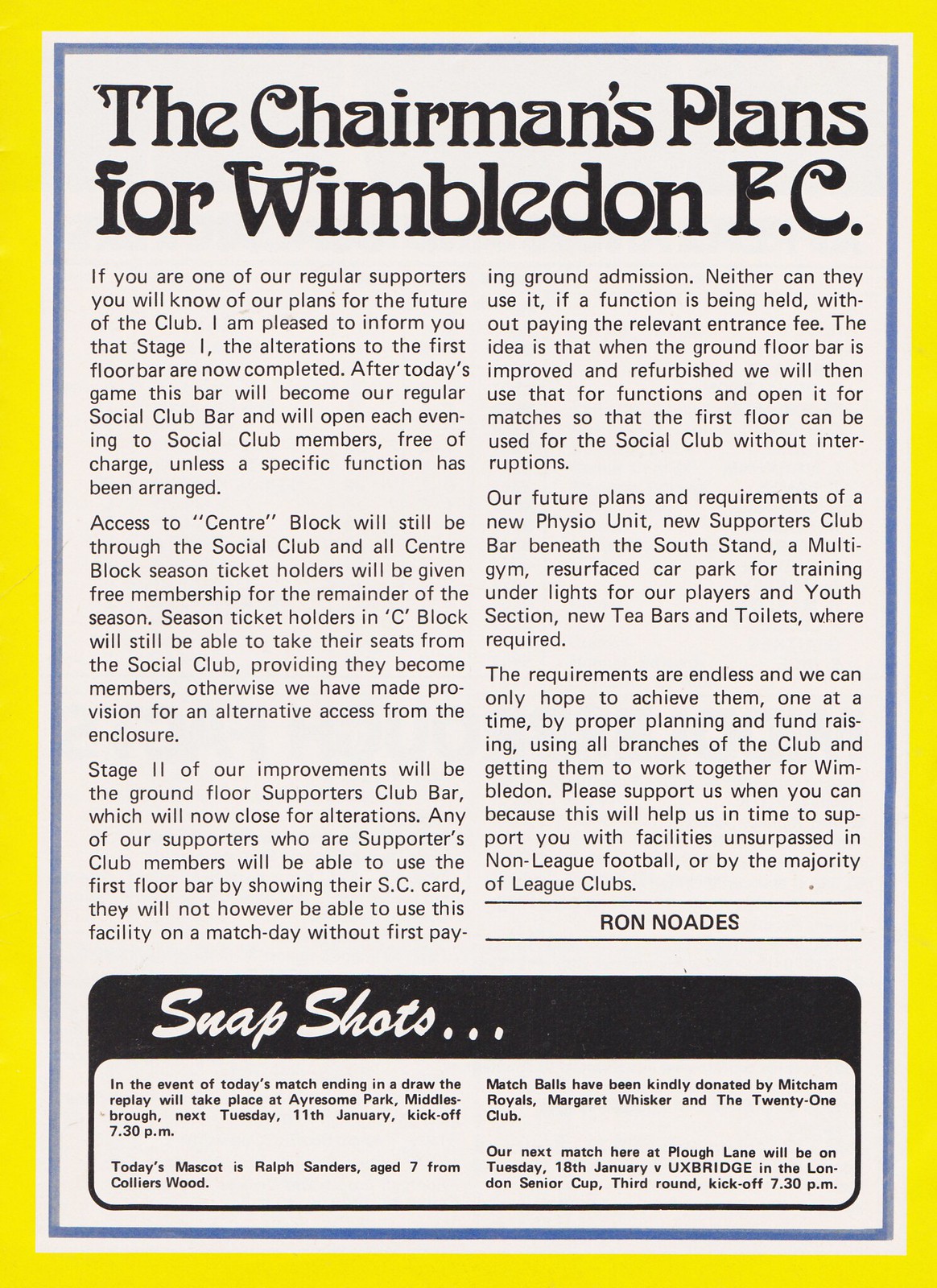This full-page advertisement, set against a gold or yellow background with a thin blue inner border, presents an important notice from the chairman of Wimbledon FC, aptly titled "The Chairman's Plans for Wimbledon FC" in bold black font at the top. The ad details the ongoing progress and future plans for the club, highlighting improvements in the facilities, access updates, and stage enhancements aimed at benefiting the club's supporters. The two columns of small print text are carefully outlined to keep the members informed and excited about the club's ongoing developments. At the bottom of the right-hand column, the plan is formally signed off by Ron Nodes in uppercase font. Additionally, below these columns, there is a sidebar labeled "Snapshots" written in white cursive font against a black border, containing an article, dated January 11th, about an event scheduled to kick off at 7:30 PM. This comprehensive ad serves both as an informative update and an encouraging message to the club's dedicated supporters, assuring them of the promising future ahead.